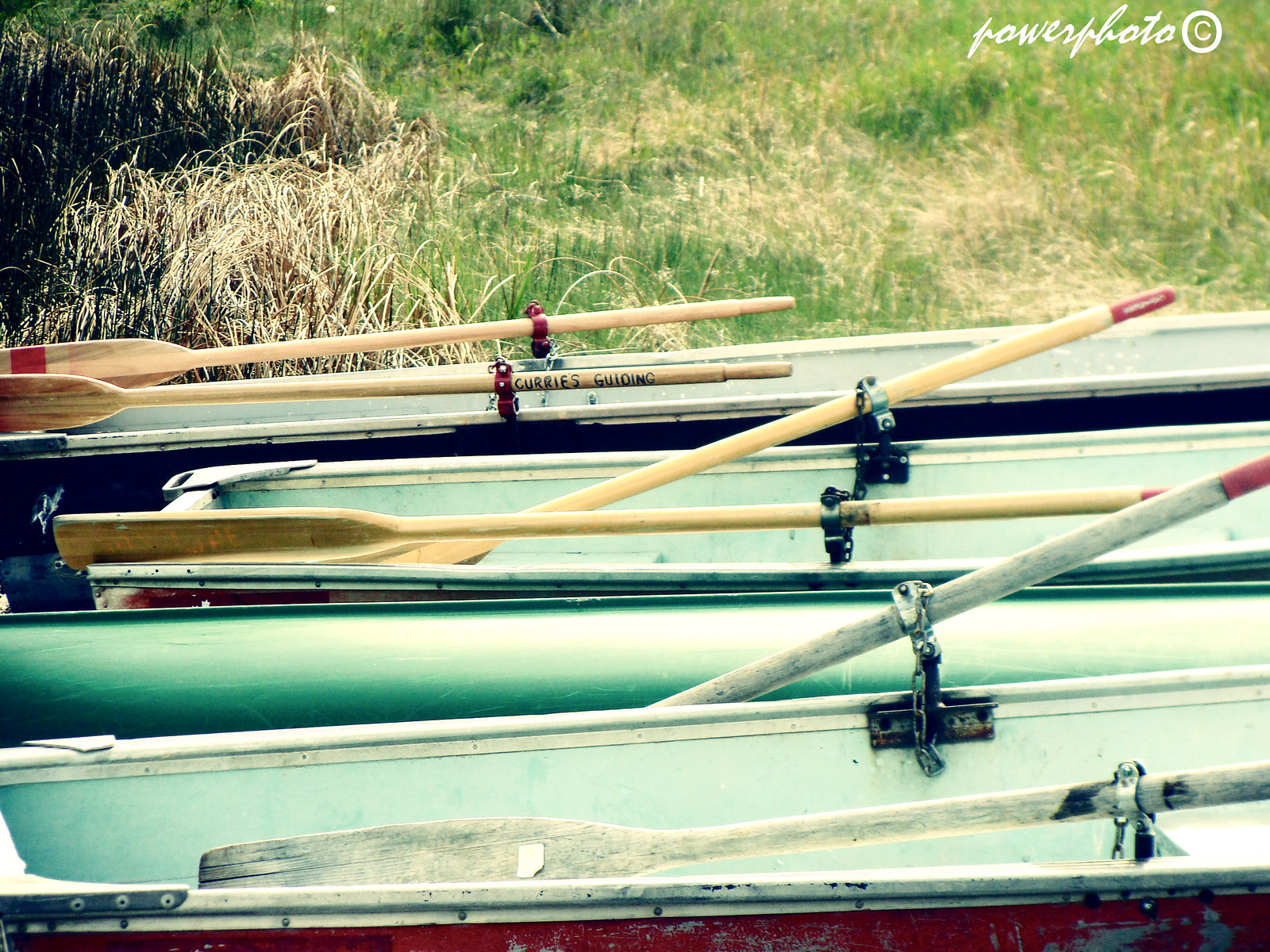This outdoor photograph captures a close-up view of four small boats, which appear to be fishing boats or canoes, lined up horizontally. The image centers on the middle sections of the boats, showing their spacious width, which could comfortably accommodate more than one person along with some supplies. The boats feature oar holders on each side to secure the oars for rowing and steering. The interior of the boats is primarily green, while the exterior is a weathered brown, although only parts of the boats' sides are visible. The first boat has a visible red or orange distressed side, and the others have varying darker hues. Oars with red tips are locked into place, with the first two being whitish and the others brown. One of the oars bears the inscription "Curries Guiding." Behind the boats lies a grassy hillside with a mix of green grass and some yellowish weeds. In the upper right-hand corner of the image, "Power Photo" is written in white script, accompanied by a © symbol.